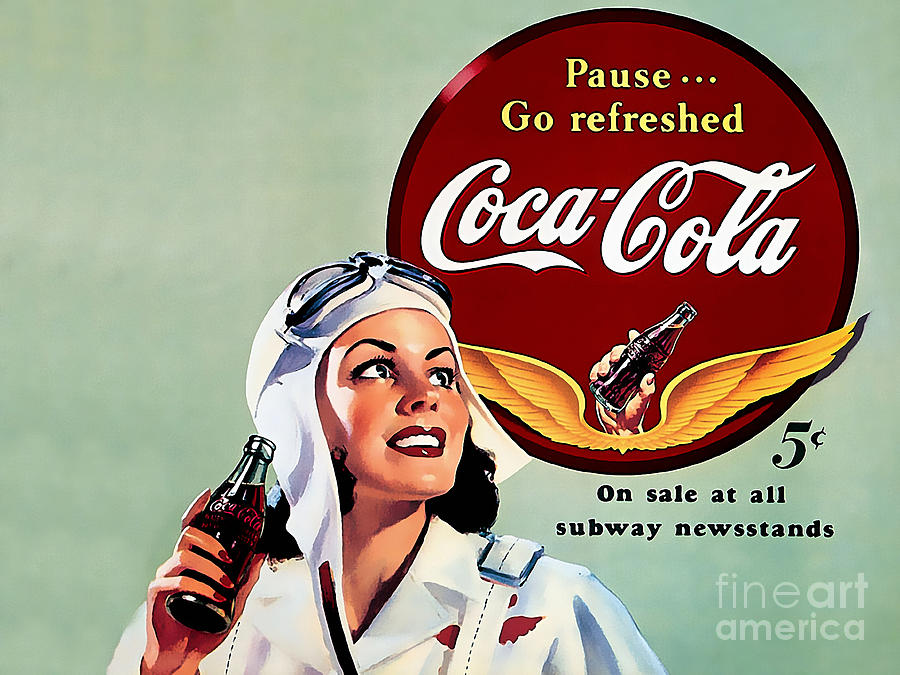This retro Coca-Cola advertisement features a pale green, cloudy background with a central image of a woman dressed as an aviator. She wears a white uniform complete with an aviator's hat and goggles atop her head, and her chest displays a set of wings. The woman, with dark hair, prominent dark eyes, red lipstick, and red fingernails, smiles broadly while holding an open glass bottle of Coca-Cola in her right hand. Above her, in a bold red circular Coca-Cola logo, the text reads "Pause, Go Refreshed, Coca-Cola." Nestled within the logo are golden wings framing a hand holding another bottle of Coke. The ad also highlights that the beverage costs five cents and is available at all subway newsstands. At the bottom corner, a watermark reads "Fine Art America."